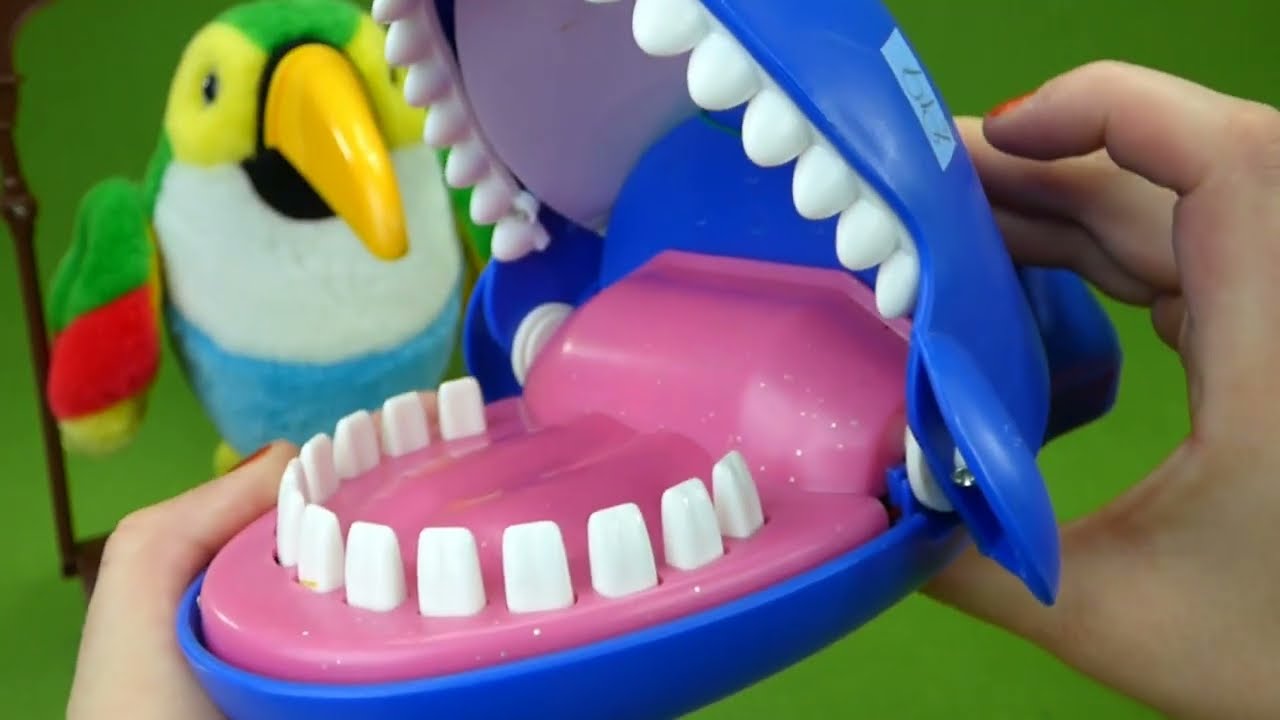The image depicts a close-up scene of a person with red nail polish on their right hand, placing a toy police car on a green ground surface. The toy police car, a black and white Tonka Rescue vehicle, features siren lights on top and the words "Police Tonka Rescue" prominently written on its side. The back of the car has the number "5147" in white font. Behind the police car, there's a large red monster truck toy with large black wheels and a smiley face decal, angled slightly backward and facing the viewer. In the background, another blue toy is partially visible. Both the surface and background of the image are green, creating a cohesive backdrop for the toys.